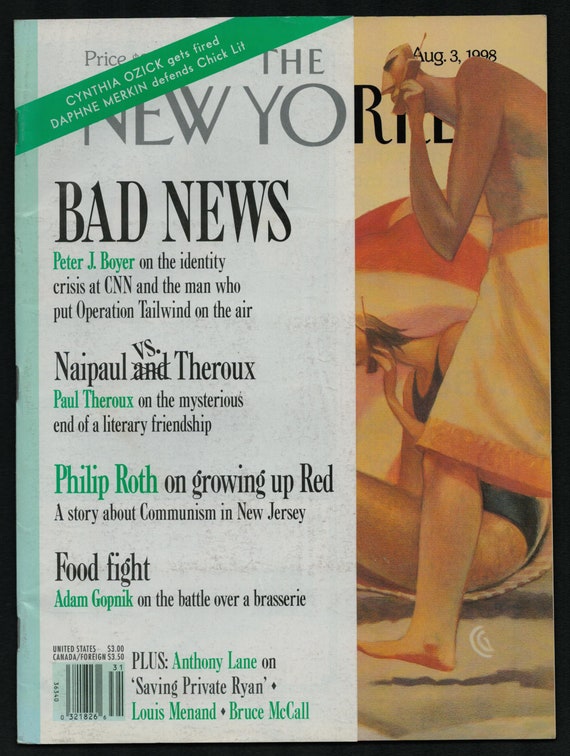This is the cover of The New Yorker magazine from August 3rd, 1998. Dominating the right third of the cover, a surreal artwork features a man with a Moai statue-like head, clutching a large, old-fashioned cell phone, and wearing swim shorts. Behind him, a woman in a black swimsuit lounges on a towel, also engaged on an antiquated cell phone. The left side of the cover is filled with headlines, all over a green backdrop. These include: "Bad News" by Peter J. Boyer on the identity crisis at CNN and the man behind Operation Tailwind; "Naipaul vs. Thoreau," Paul Theroux delves into the mysterious end of a literary friendship; "Philip Roth on Growing Up Red," a narrative about communism in New Jersey; and "Food Fight," Adam Gopnik discusses the battle over Brasserie. Additional mentions include Anthony Lane on "Saving Private Ryan," Louis Menand, and Bruce McCall. The barcode is positioned at the lower left corner, marking it as a classic 1998 issue.